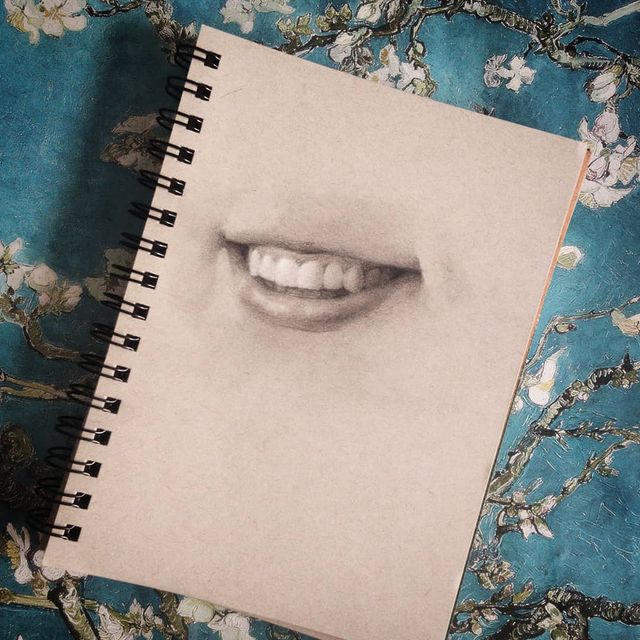The image depicts a large square picture of a spiral notebook placed diagonally with the black spiral binding on the left side. The notebook has a light gray or white cover featuring a detailed drawing of a smiling mouth with perfectly white teeth and glossy lips. The mouth illustration includes the upper lips slightly and a more prominent depiction of the lower lips. The background on which the notebook rests is a vibrant blue tablecloth adorned with white flowers attached to vines that extend from the right upper corner as well as the lower right and left corners. The overall image is brightly lit, clear, and captures the intricate details of both the notebook and the floral background.